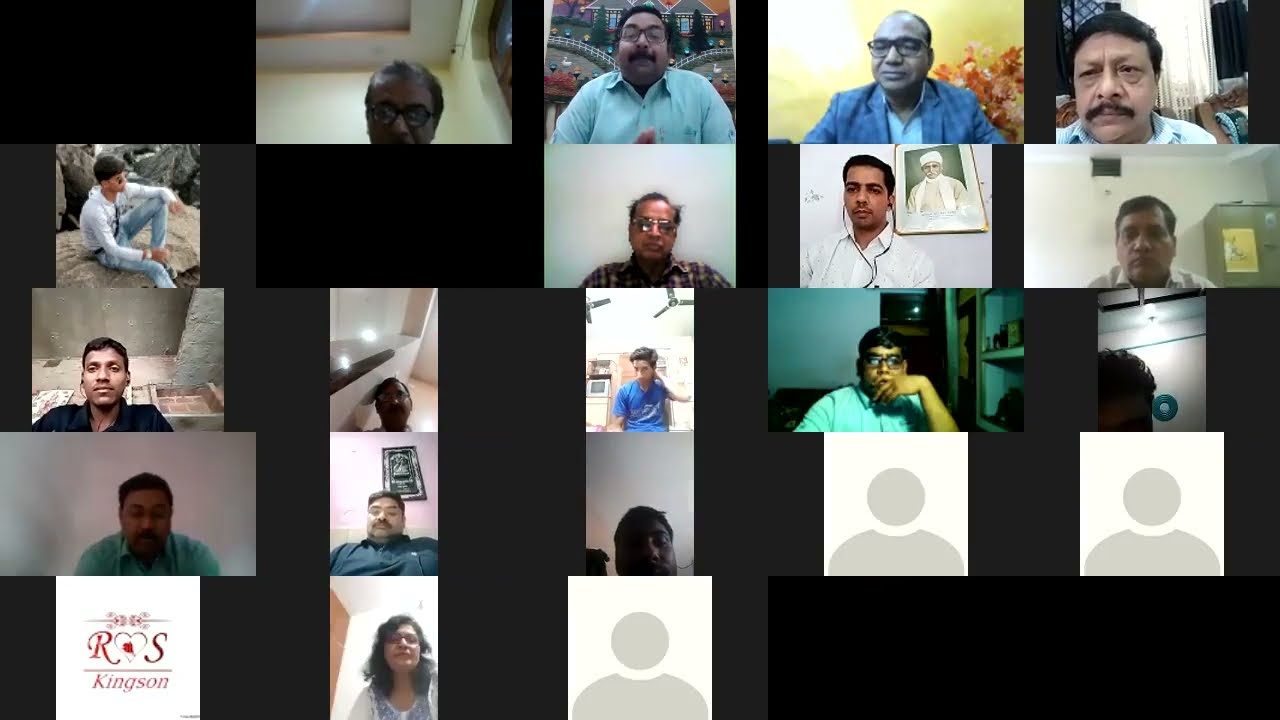The image resembles a Zoom meeting grid with multiple smaller boxes within a larger one, each displaying a different person, mostly Indian men, with one woman. The setting looks like a screen grab from an online session with 23 visible participants, each in varying states of engagement. 

In the first row of four figures, we see:
1. A man wearing glasses, captured mostly from the mustache up.
2. Another man in a teal shirt, hands clasped together, also wearing glasses and sporting a mustache.
3. A man in a buttoned jacket with a yellow background, clean-shaven and wearing glasses.
4. An older man with a mustache and no glasses, close to the camera.

The second row contains:
1. An image of a man on a rock in blue jeans, long-sleeved shirt, and sunglasses.
2. A black box with no visible person.
3. A man in a black and brown plaid shirt with uncombed hair and glasses.
4. A man in a white button-up shirt, wearing headphones, with a portrait visible behind him.
5. Another man in a white button-up shirt with poor lighting, appearing slouched.

The third row features:
1. A man in a black button-up shirt, wearing headphones, with a hint of a brick background.
2. A man poorly lit, with a single shining light and white walls in the background.
3. A man in a blue shirt, one hand behind his neck.
4. A man in a teal button-up shirt, wearing reading glasses.
5. A man poorly lit, barely an outline of his face visible.

The bottom row includes:
1. A man in a teal shirt with a white background, face obscured by lighting.
2. A man in a black polo, viewed from the belly button up, sporting a mustache.
3. A man close to the camera, seen from an odd angle, almost looking up his nose.
4. Two blank photo boxes showing the default silhouette of a person.

Below these rows:
1. An avatar icon with text saying "R. Hart S. Kingston."
2. A woman with shoulder-length hair in a white and blue shirt.
3. Another avatar icon for someone present but not sharing their video.

The overall composition and varying backgrounds, attire, and lighting in this grid of faces reflect a diverse, real-time virtual meeting or class in progress.